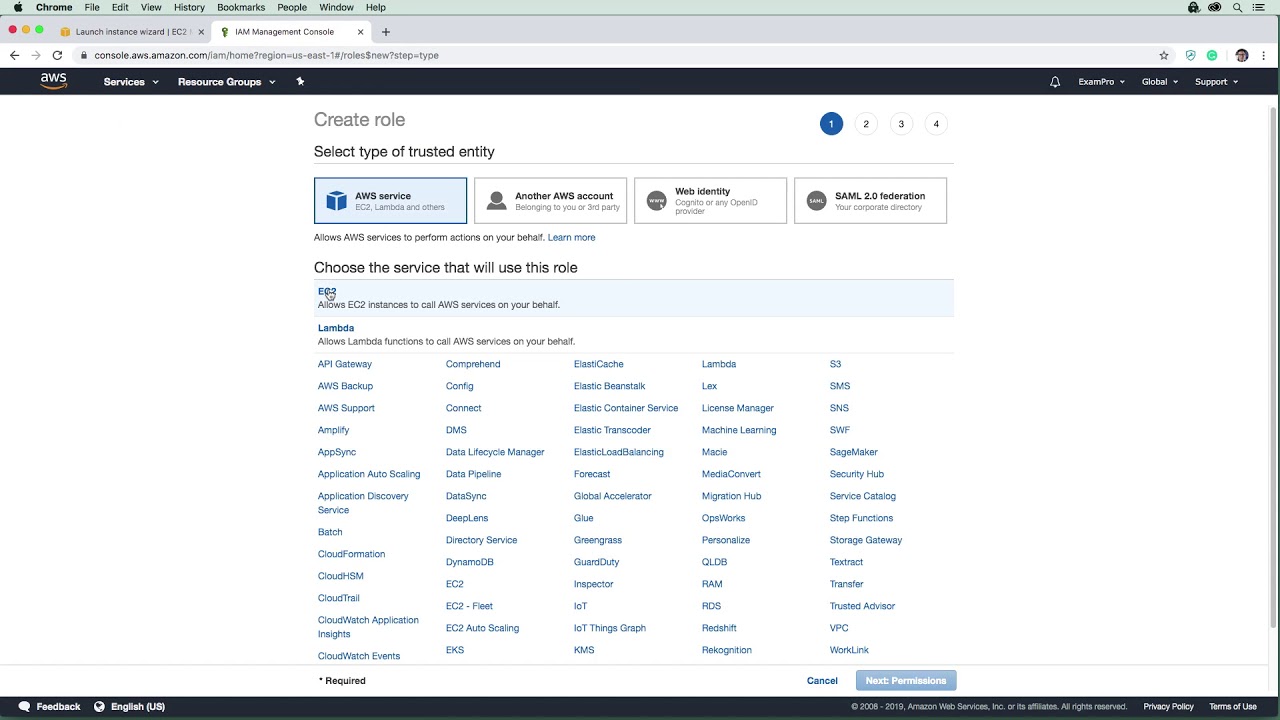The image appears to be a screenshot taken of a computer screen using a device that runs on macOS, indicative of a MacBook or iMac. The screenshot captures an activity on the AWS Management Console's Identity and Access Management (IAM) page. The specific URL visible in the screenshot is "https://console.aws.amazon.com/iam/home?region=us-east-1#roles$new?step=type".

The header section of the webpage features a distinct black bar that includes the AWS logo on the left, a dropdown menu for 'Services', an option for 'Resource Groups', and a pin icon. To the right of the header, there are several icons and dropdowns: a bell icon for notifications, a link labeled 'Exam Pro', a 'Global' selector likely for region settings, and a 'Support' dropdown.

Dominating the main view of the page is the role creation interface, starting with a prompt to create a new role. This section is set against a clean, white background. Users are given the option to select the type of entity for which they are creating the role, with choices including 'AWS service', 'Another AWS account', 'Web identity', and 'SAML 2.0 federation'. Below this selection area is an extensive list of AWS services, each hyperlinked in blue, enabling user interaction and selection.

At the bottom of the screen, there are options for providing feedback and changing the language. The bottom navigation bar also includes a 'Next' button, suggesting that this is part of a multi-step process on the IAM console for creating a new role.